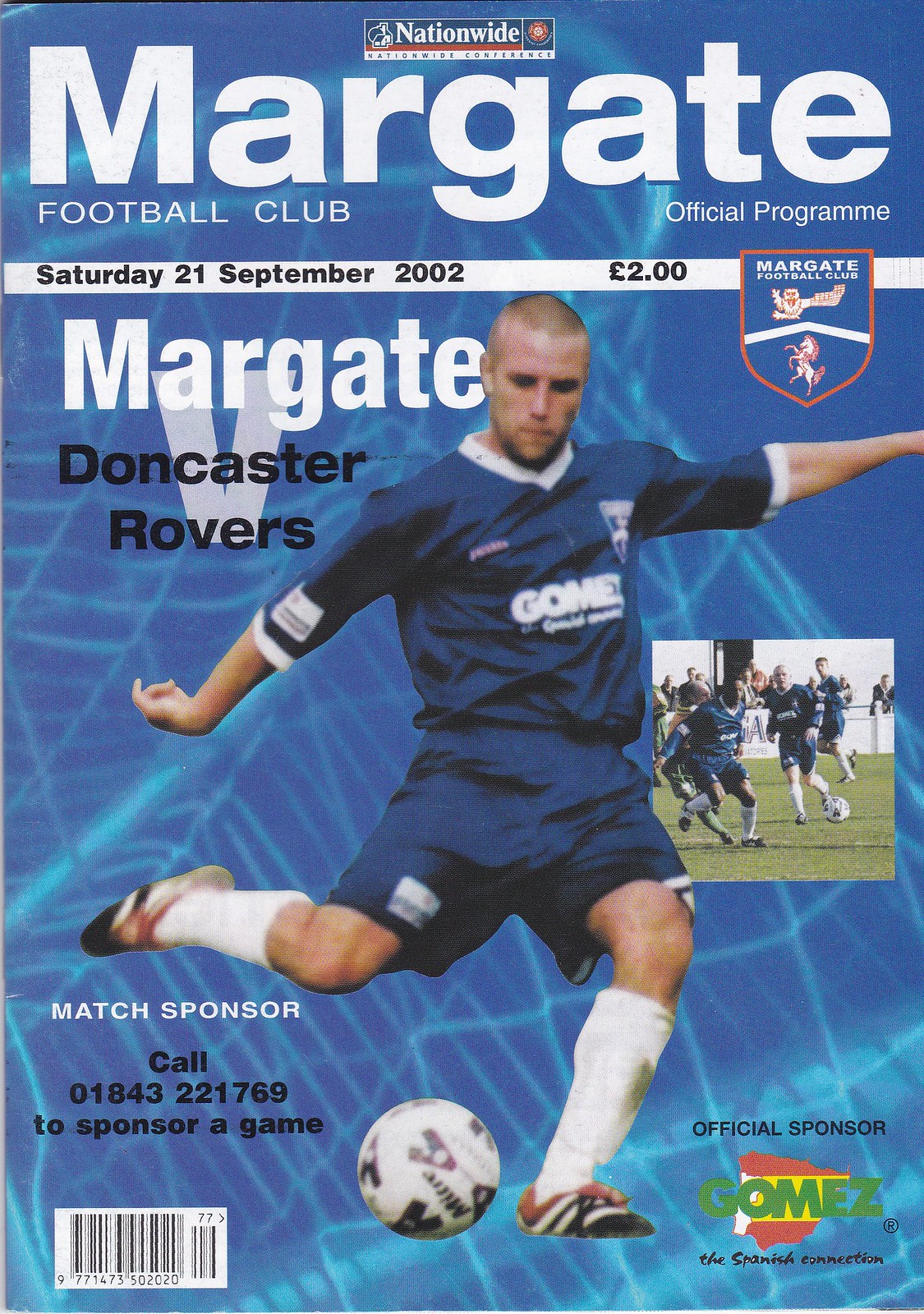The front cover of the Margate Football Club magazine for Saturday, September 21st, 2002, priced at £2, features a striking design with a blue background adorned with an abstract lighter blue net pattern. At the top, the Nationwide logo in blue and red with white lettering sets off the cover. Dominating the page, the word "Margate" stretches in bold white text, with "Football Club Official Program" positioned just below. A narrow white band along the top displays the date, "Saturday, 21 September 2002," and the price, "£2," in black text, adjacent to the Margate Football Club's shield logo, depicting a red horse on a blue background.

Central to the cover is an image of a soccer player with a shaved head, wearing a blue uniform with the word "Gomez" visible, symbolizing the unofficial sponsor, the Spanish Connection. The player is captured mid-action, kicking a soccer ball, with a boxed overlay of an active soccer match. The match details, "Margate vs. Doncaster Rovers," are prominently displayed in white text beneath the club logo. The cover features the prompt to contact 01843-221-769 to sponsor a game, reinforcing the match sponsor message alongside the image. The magazine's blue and white color scheme creates a cohesive and vibrant look for the Margate Football Club's official program.